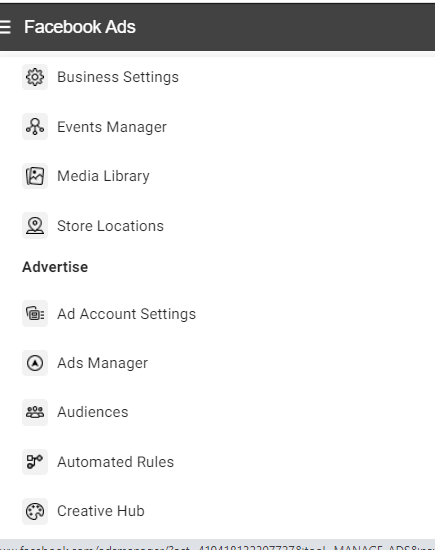This black-and-white image is a screen capture of Facebook's ads menu. Dominating the top of the image is a black bar with the words "Facebook Ads" prominently displayed in white letters. Directly below this header is a comprehensive list of menu options for configuring and managing Facebook advertisements.

The topmost menu item is "Business Settings," providing essential controls for overarching business management within the Facebook ads ecosystem. Following this is the "Events Manager," designed for tracking and managing conversion events, a critical tool for performance analysis.

Next, we encounter the "Media Library," a repository for storing and organizing all media assets like images and videos used in ad campaigns. "Store Locations" appears beneath it, offering functions to manage and promote physical store locations through Facebook ads.

The subsequent section labeled "Advertise" includes several sub-options: first is "Ad Account Settings," the hub for financial and administrative controls of advertisement accounts. This is followed by "Ads Manager," an interface for creating, editing, and analyzing ad performance.

The menu continues with "Audiences," a feature for creating and managing target audience groups, crucial for precise ad targeting. "Automated Roles" comes next, providing templates and automation tools to streamline ad production and management processes, and lastly, the "Creative Hub," a collaborative space for developing and testing ad creatives before they go live.

Every item listed in this menu is a fundamental component in the toolkit for creating, deploying, and monitoring effective and engaging Facebook advertisements.